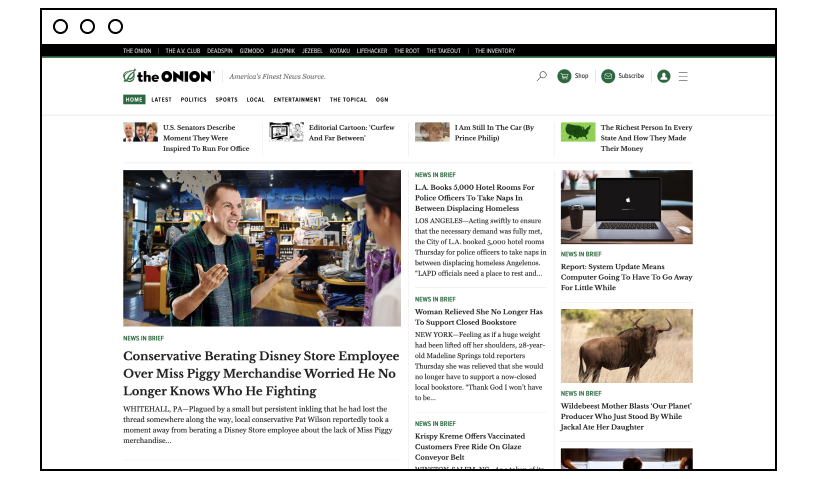The image depicts a detailed view of a satirical news website, prominently displaying the logo and motto of "The Onion: America's Finest News Source" at the top. Accompanying the logo is an illustration of a green onion cut in half. Below this, the website features navigation tabs for various affiliated sites, including The A.V. Club, Deadspin, Gizmodo, and Jezebel, indicating a network of related content.

The central portion of the webpage showcases a series of humorous and satirical headlines. Some examples include:
- "U.S. Senators Describe Moment They Were Inspired to Run for Office"
- "Editorial Cartoon: Curfew and Far Between"
- "I'm Still in the Car by Prince Philip"
- "The Richest Person in Every State and How They Made Their Money"

Taking center stage in the main section is an article featuring a photograph of a man inside what appears to be a Disney store. The man, with an animated expression and hands gesturing outward as if questioning, is facing another individual. The accompanying headline humorously reads: "Conservative Berating Disney Store Employee Over Miss Piggy Merchandise No Longer Knows Who He's Fighting." This headline indicates a comedic, exaggerated scenario of a disgruntled customer in a Disney store.

Further down the page, another headline satirically notes, "L.A. Books 5,000 Hotel Rooms for Police Officers to Take Naps in Between Displacing Homeless," showcasing the site's penchant for blending humor with pointed social commentary.

Overall, the website employs a mix of comedic and surreal content, characteristic of The Onion's well-known satirical style.